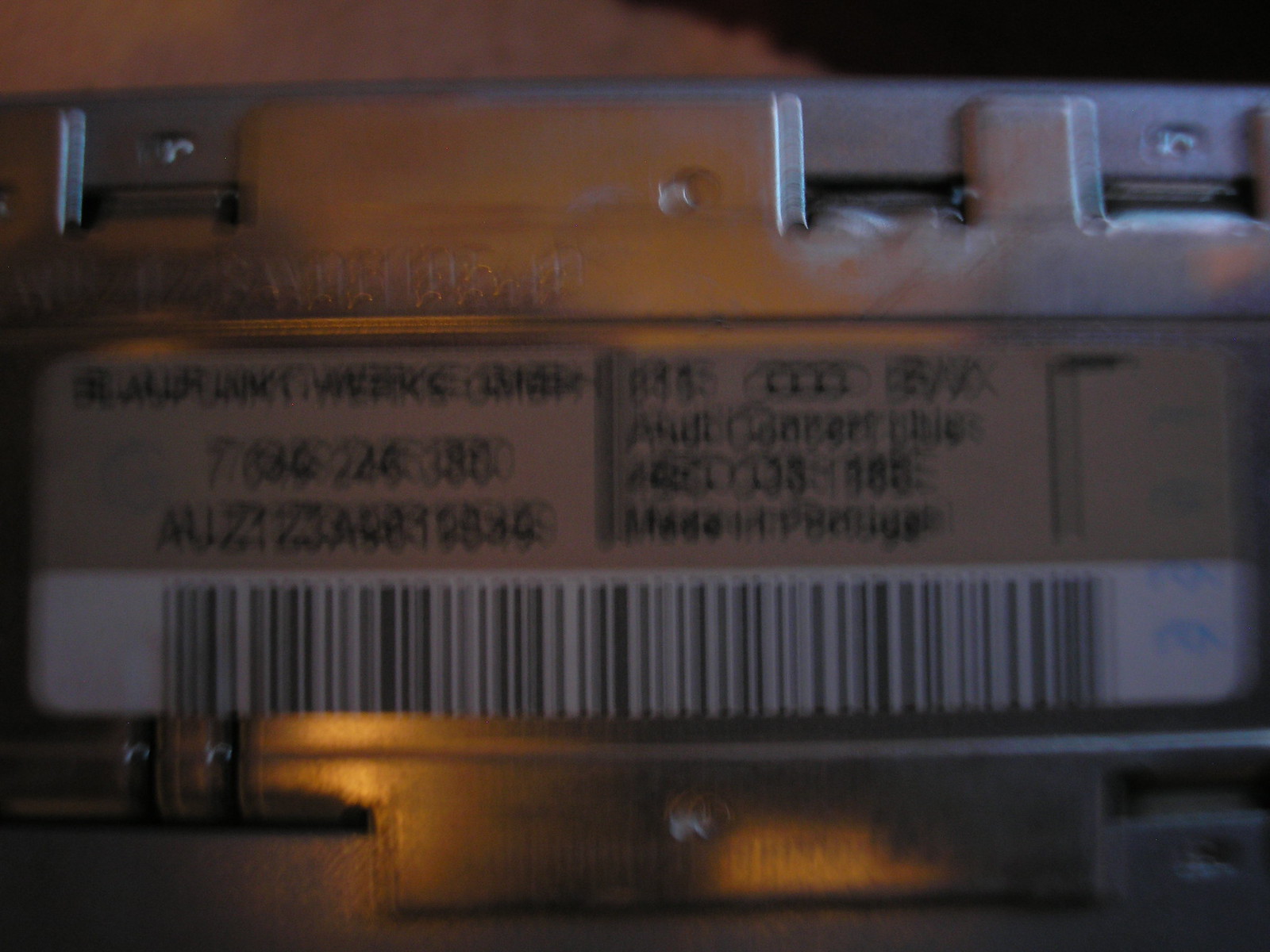This photograph presents the unclear, underside view of a large object with a gold metallic hue. In the center, there is a series of black alphanumeric characters, although they are too blurry to be distinctly identified. Below this series is a sizable white rectangle outlined with black dashed lines. The overall image has a washed-out appearance, with significant light reflections adding to the general blurriness, making it challenging to discern any specific details. The object appears to have a large surface area, contributing to the impression of its substantial size.